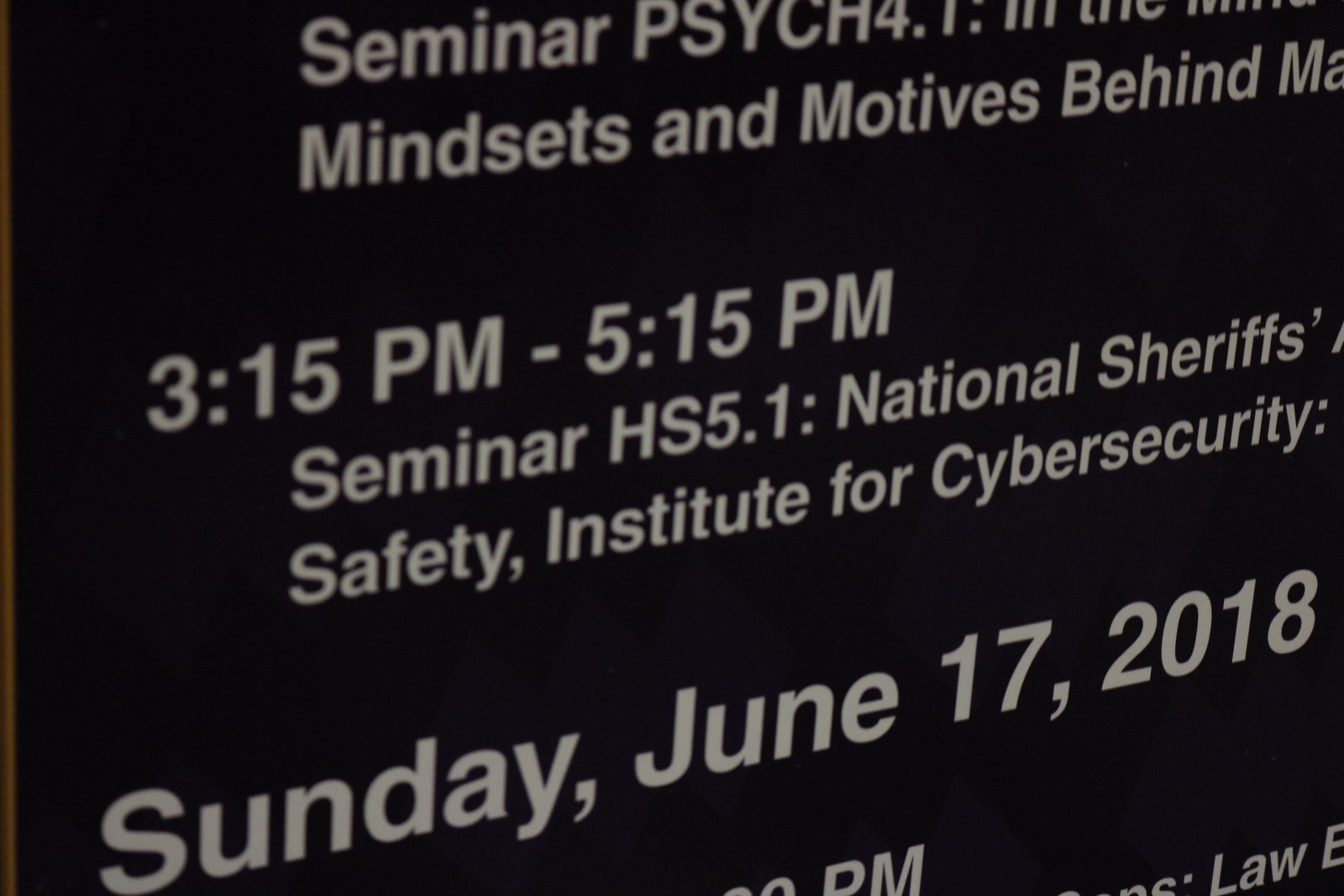The image features a black background with white text, which appears slightly blurred at the top. The text is arranged in multiple lines, suggesting it could be part of a larger sign or a screen, possibly an announcement for a seminar or conference. The visible text reads: "Seminar Psych 4... Mindsets and Motives Behind..." followed by the details "3:15 to 5:15 PM, Seminar HS 5.1, National Sheriff's Safety Institute for Cyber Security." The date on the sign is prominently displayed as "Sunday, June 17th, 2018." The image seems to capture only a portion of the full announcement, with some text cut off, indicating different seminar sessions scheduled close together. The overall style suggests an organized schedule of events, possibly for a conference or educational seminar series.